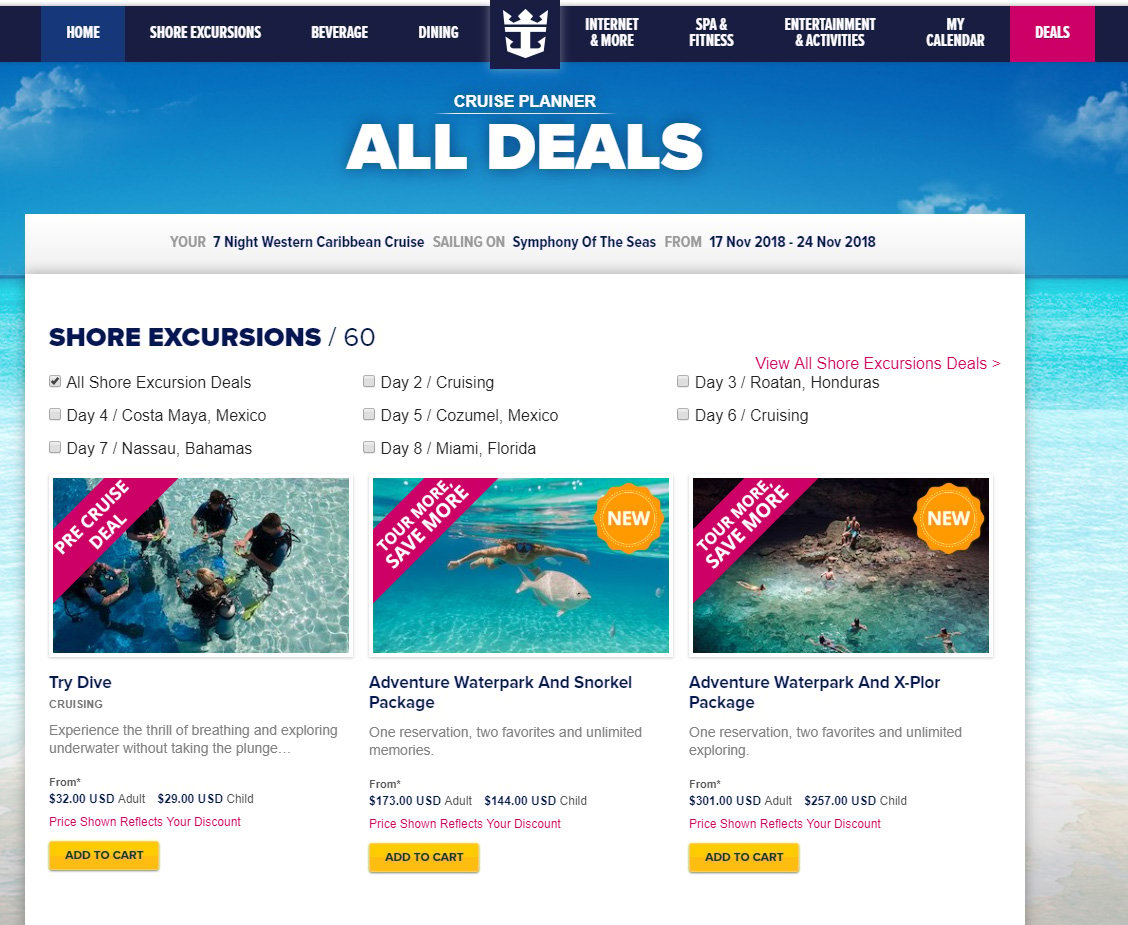The image depicts a cruise planner interface highlighting all available deals in a clean, white-themed layout. At the top center, a prominent anchor symbol adorned with a crown represents the cruise brand. Surrounding the logo are navigational tabs leading to various sections of the site: Home, Shore Excursions, Beverage, Dining, Internet and More, Spa and Fitness, Entertainment and Activities, My Calendar, and a pink-highlighted Deals section.

The background features a serene illustration of a clear blue sky merging with the ocean and shoreline, creating a tranquil atmosphere. In the main white section of the page, the text states: "Your Seven-Night Western Caribbean Cruise sailing on Symphony of the Seas from 17 November 2018 through 24 November 2018."

Beneath this information, the section shows details about available shore excursions, listing 60 options. Highlighted excursion details for stops like Costa Maya, Mexico on Day 4 and Nassau, Bahamas on Day 7 are presented. Below this, there are colorful thumbnails representing various activities. 

- The first thumbnail depicts divers exploring underwater, suggesting a diving excursion.
- The second thumbnail features a person swimming with a sea creature, hinting at a marine life encounter.
- The third thumbnail showcases a group of people in a cave, indicating a caving adventure.

Each thumbnail includes a brief description, the activity's price, and a prominent yellow "Add to Cart" button for easy purchase. The overall design is user-friendly, visually appealing, and focuses on engaging the viewer with detailed activity options.